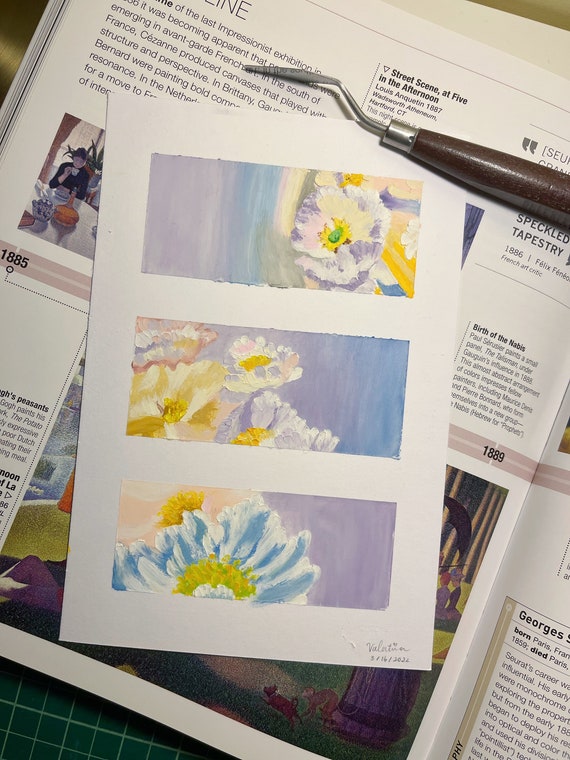In this detailed image, you are seeing an open magazine or book placed on a green grid background. The magazine page, possibly a historical or art-related publication, includes dates like 1885 and 1889 and phrases such as "street score at fire to the afternoon" and "street scene." Lying across the top right corner of the magazine is a silver tool with a metal bar leading to a wooden handle. Centered on top of this magazine is a rectangular sheet of white cardstock paper, which features three vertically aligned pastel watercolor paintings. Each rectangle contains a depiction of daisies, characterized by yellow, blue, and white flowers, set against soft hues of blue, purple, green, and yellow. The artist’s name and the date of creation are noted at the bottom right of the card. The entire setup, with its professional and aesthetically pleasing arrangement, exudes a sense of artistic appreciation and meticulous composition.